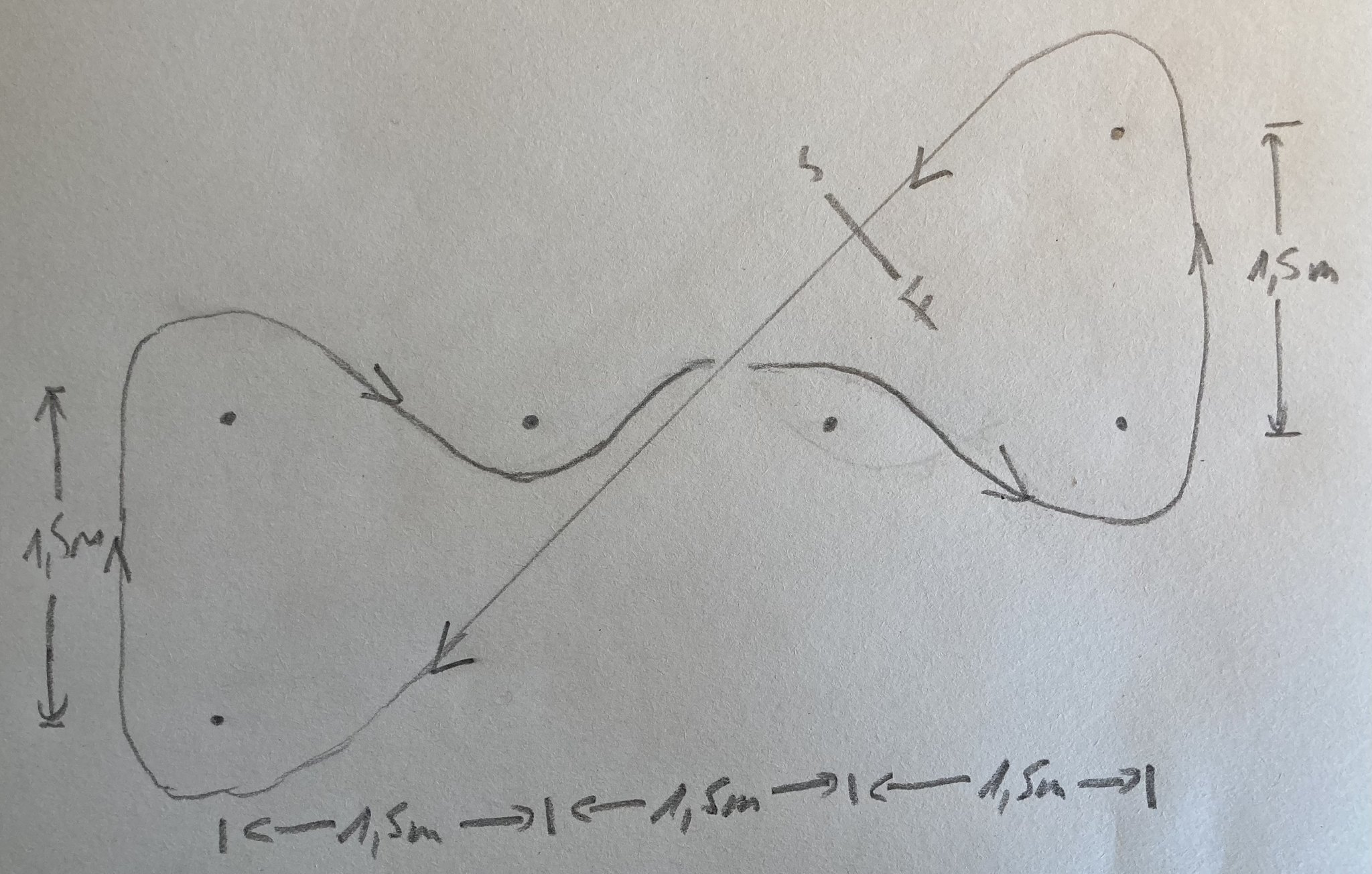The image depicts a detailed hand-drawn diagram on standard white computer paper. Central to the drawing is a prominent infinity symbol, constructed from arrows, evoking the sense of continuous or cyclical motion. Within this infinity loop, letters "F" and "S" are positioned across from each other, suggesting opposing or complementary elements. Below the infinity symbol, additional arrows are marked with letters "A" and "S," possibly indicating steps or stages within a process. On the left side of the paper, two arrows point away from each other, adorned with the letters "S" and "M," which may signify divergence or balance between two entities. The minimalist yet thoughtfully structured nature of the diagram suggests a conceptual framework, perhaps for a process, cycle, or system.